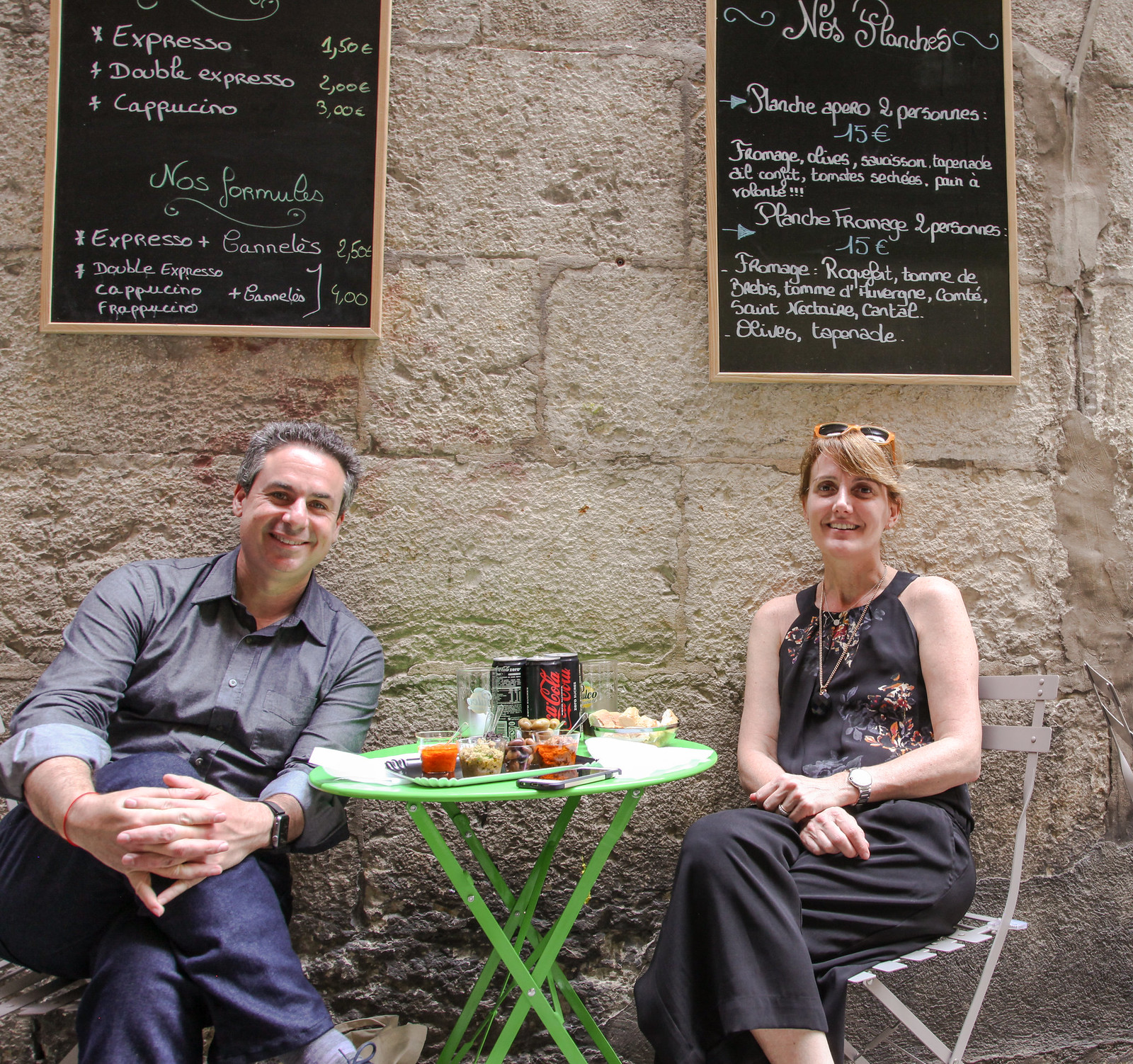This image depicts two people seated at a small, round, light-colored outdoor table, located outside a rustic building with a stone wall. Behind them, two black chalkboard menus are mounted on the wall, listing items such as espresso, double espresso, and cappuccino, with prices written in both white and occasional green or blue chalk. To the left side of the table, a man with short, slightly graying dark hair, dressed in a gray long-sleeved shirt and blue jeans, sits with his legs crossed and his hands folded in front of his knee. On the table, various items are visible, including a tray holding assorted food items, a few beverage cans including Coca-Cola, and a phone. Seated to the right of the table, a woman with short, blondish hair adorned with sunglasses perched on top, wears a black floral dress and a necklace, with her arms resting on her lap. She appears to be looking slightly upward and to the left, while facing forward. This scene, possibly set in a European locale like France or Italy, captures a relaxed moment as the pair share a meal outdoors.